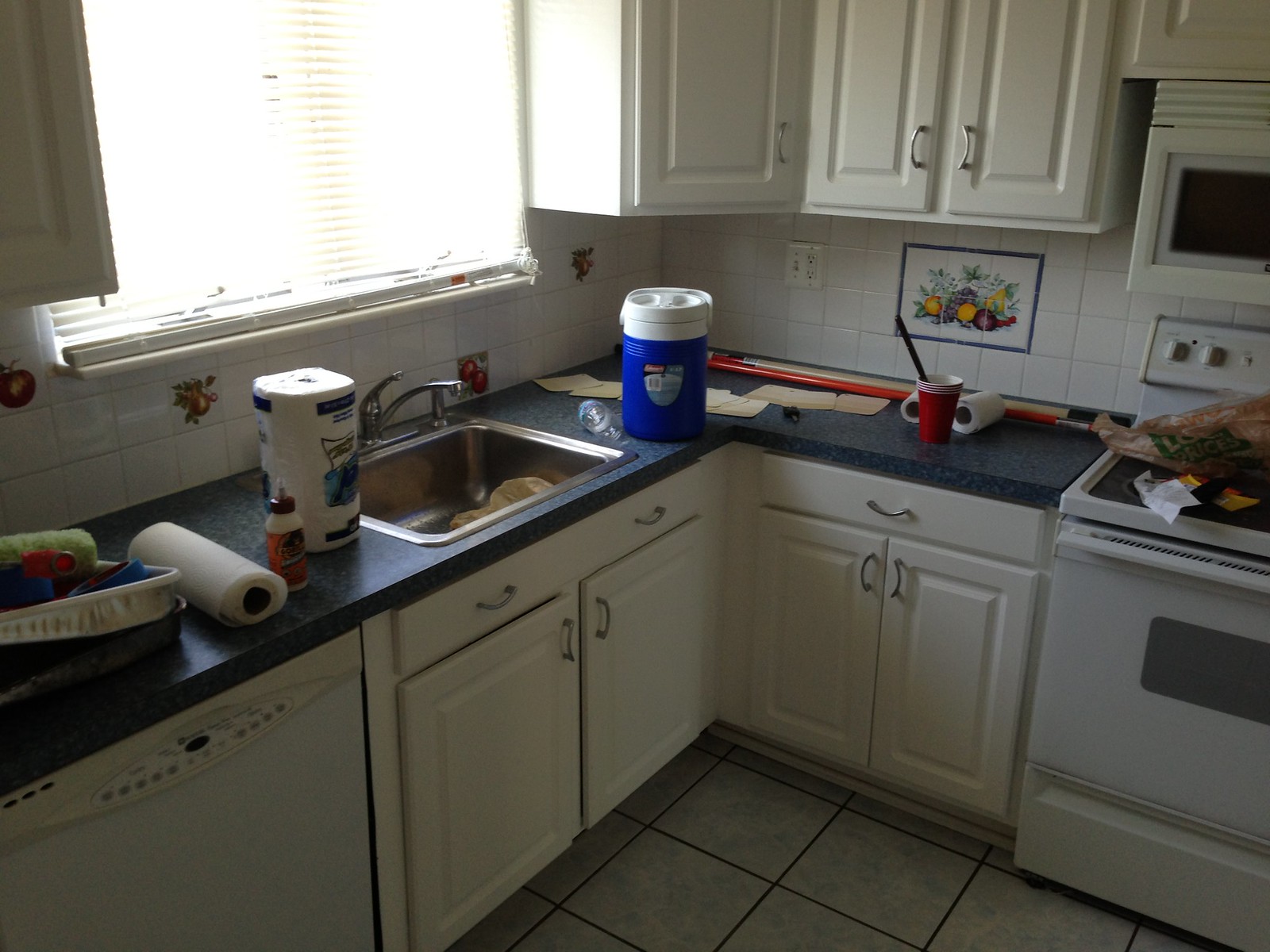This photograph, taken at standing height, offers a detailed view of an L-shaped kitchen from the perspective of someone standing within it. The kitchen features dark-colored laminate countertops, with a stainless steel sink prominently located at the juncture of the L. Within the sink, a sponge can be observed.

In the lower left corner of the image, a washing machine is partially visible. Next to it, a series of under-sink cabinets run along the left section of the counter. The right side of the L-shaped configuration houses additional cabinets, an oven, and a range with a sleek, flat glass surface. Above the countertop, there are more cabinets, including a microwave situated above the stove. Between the upper cabinets and directly above the sink, a large window allows natural light to fill the space.

The countertop is cluttered with various items. To the left of the sink, there is an unwrapped roll of paper towels lying on its side and another, still wrapped, standing upright. To the right of the sink, a blue cylindrical thermos cooler and an empty water bottle are present. Nearby, a few red cups suggest that some sort of home improvement activity, possibly painting, is underway. Adding a touch of charm to the space, the tiles next to the stove feature a small painted tableau of fruits and vegetables.